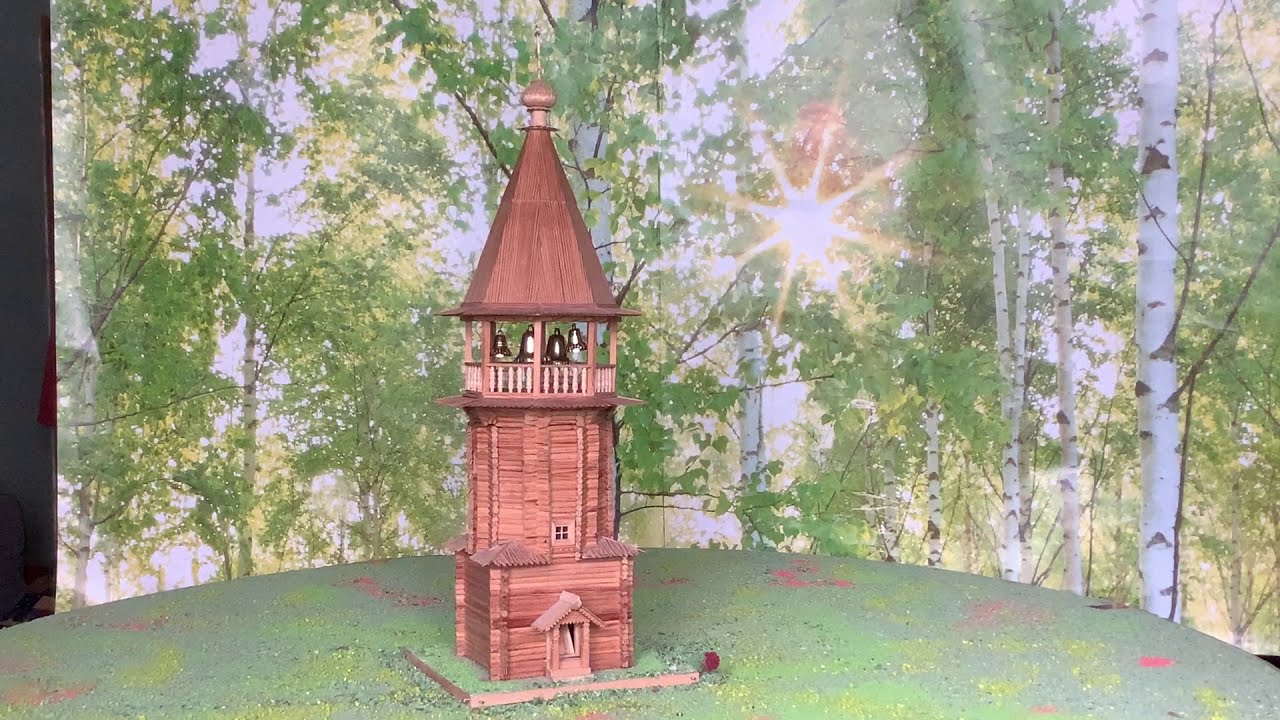The photograph depicts a detailed, hand-crafted model of a tall, log-cabin-style church made from thin wooden sticks or tongue depressors. The structure includes a cone-shaped steeple or bell tower that houses four copper-colored bells. The base of the model sits on a wooden platform, intricately decorated with green paint and specks of yellow and red glitter. This platform is placed on a table adorned with a tablecloth. The background of the image features what appears to be a forest of tall aspen trees with sunlight filtering through, suggesting an artificial backdrop rather than a real outdoor scene. The model includes a small door, and the backdrop has elements of photo manipulation, adding to the overall picturesque and rustic aesthetic of the scene.